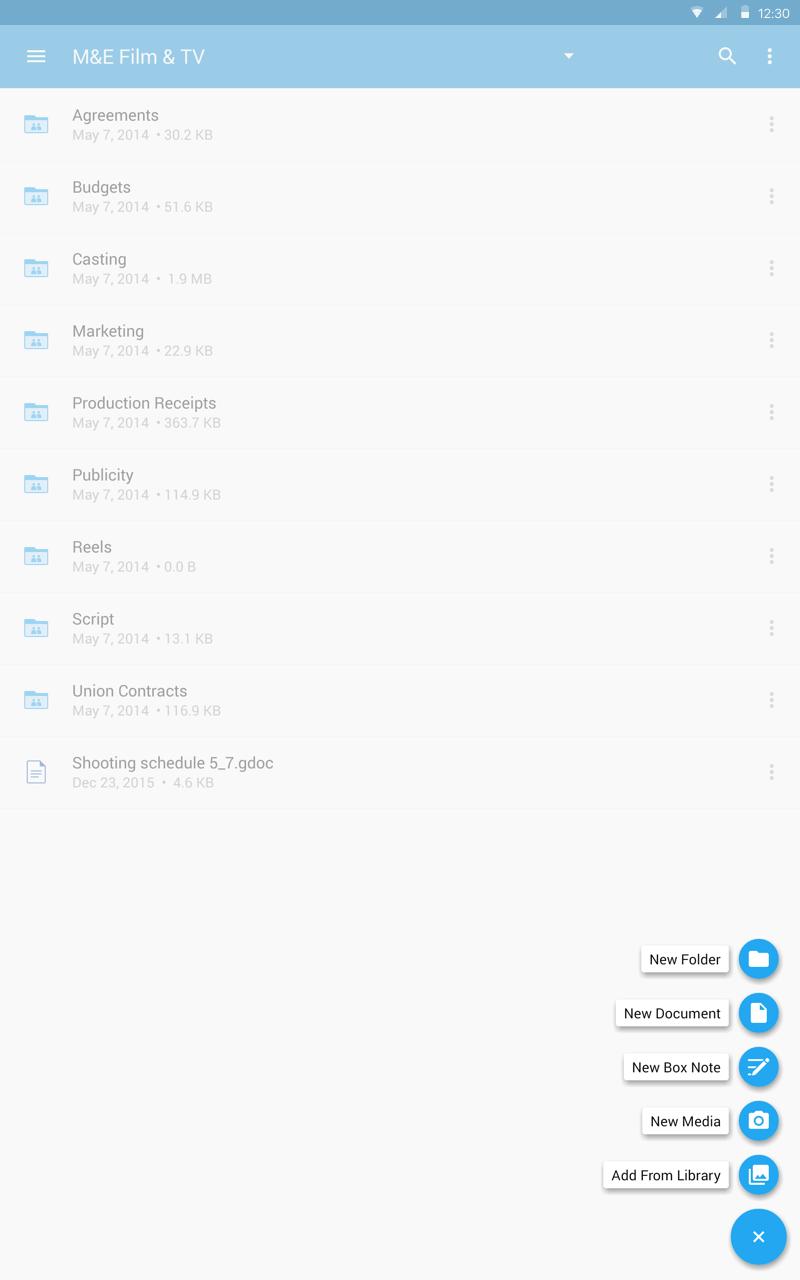This detailed image caption describes a screenshot from the MNE Film and TV website. The screenshot features a blue header and a list of items, each with descriptive text and file sizes. The list includes:

1. **Agreements** - Posted on May 7, 2014, at 30.2 kilobytes.
2. **Budgets** - Posted on May 7, 2014, at 51.6 kilobytes.
3. **Casting** - Posted on May 7, 2014, same date.
4. Additional items such as **Marketing**, **Production Receipts**, **Publicity**, **Reels**, **Script**, **Union Contracts**, and lastly, 
5. **Shooting Schedule 5_7.doc** - Posted on December 23, 2015.

The first set of items features a blue folder icon next to them, while the **Shooting Schedule 5_7.doc** has a document icon. 

On the bottom right of the screenshot, there are several icons contained within blue circles, each representing different actions:
- **New Folder** - Depicted with a file icon.
- **New Document** - Depicted with a white page icon.
- **New Box Note**.
- **New Media** - Depicted with a camera icon.
- **Add from Library** - Depicted with two overlapping documents.

There's also an icon featuring a blue circle with an 'X' at the bottom, which presumably indicates the action to close or delete. 

All these icons and their associations are aligned on the left side of each item title, providing a clear and organized representation of various file types and actions available on the MNE Film and TV platform.